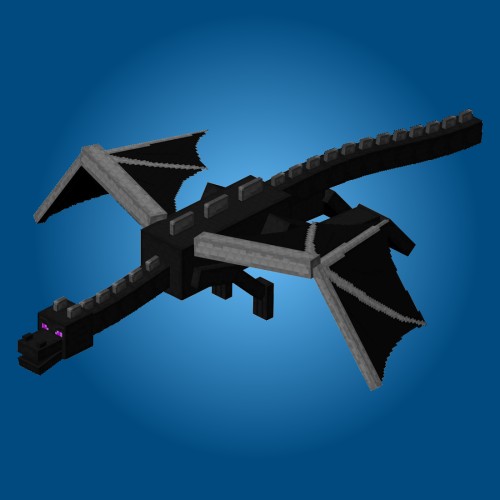The image showcases a black dragon constructed from Legos or a similar block-based medium, characterized by its blocky, 8-bit nature reminiscent of Minecraft graphics. The dragon features a predominantly black body, tail, and head, accentuated with gray or silver scales along its back and the front part of its wings. These wings, like the rest of the dragon, exhibit a rectangular and square geometry, contributing to an overall very blocky aesthetic. The dragon has striking pink eyes that stand out against its dark body. In the background, a spotlight illuminates the dragon, casting it into sharp relief against a gradient blue backdrop that transitions from darker blue at the edges to lighter blue towards the center, suggesting motion and an aerial scene. The dragon appears to be in mid-flight, positioned centrally within the image, evoking a sense of dynamic movement.